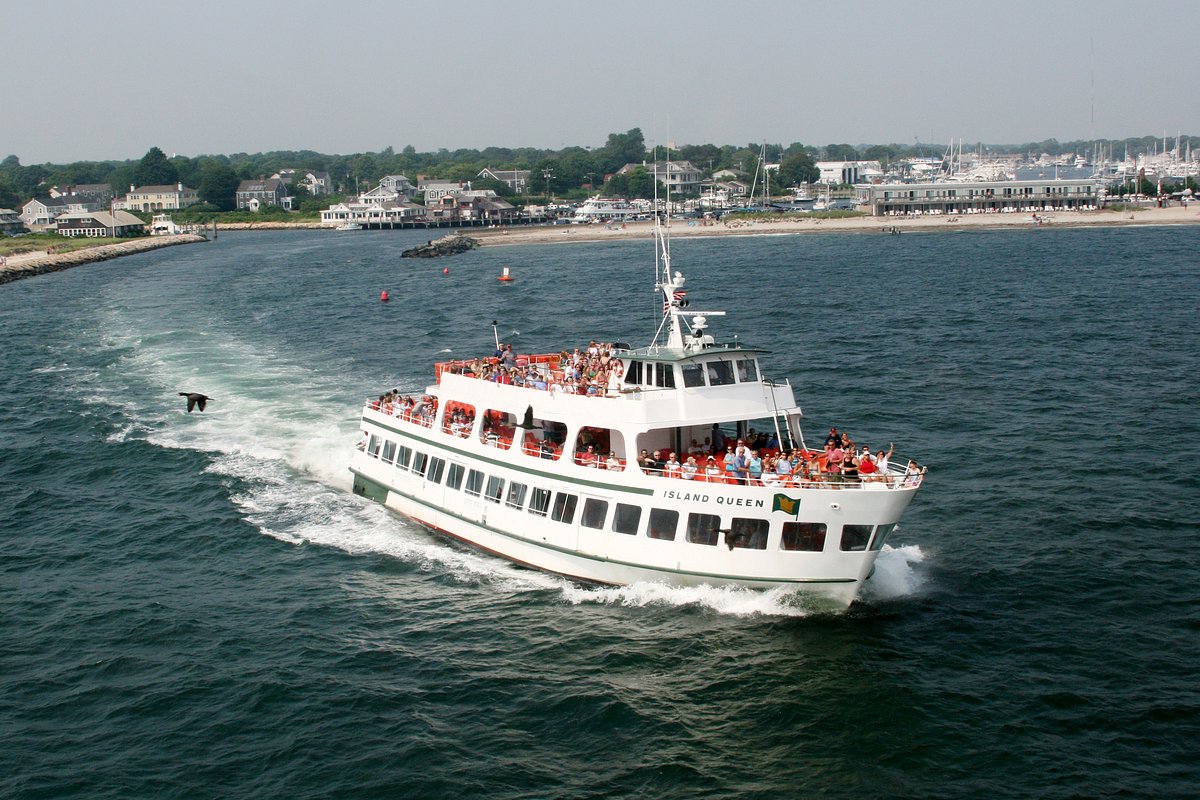This vibrant daytime photograph captures a serene waterscape featuring a large, white boat named "Island Queen," adorned with green trim and a flag bearing a gold crown. The two-deck boat, populated with people enjoying the view, is navigating away from the shore, leaving a visible wake in its path. Above, a bird soars through the beautifully blue sky, adding to the lively atmosphere. Closer to the shore, three orange buoys float, and a rocky pier extends into the water. In the backdrop, several homes with green lawns and trees stand along the shore, hinting at a charming village or town setting. To the right, a marina features numerous sailboats, some docked and some gently swaying in the water. The overall scene is characterized by abundant greenery, clear sunlight, and a picturesque harbor, reflecting a day of leisure and scenic beauty.